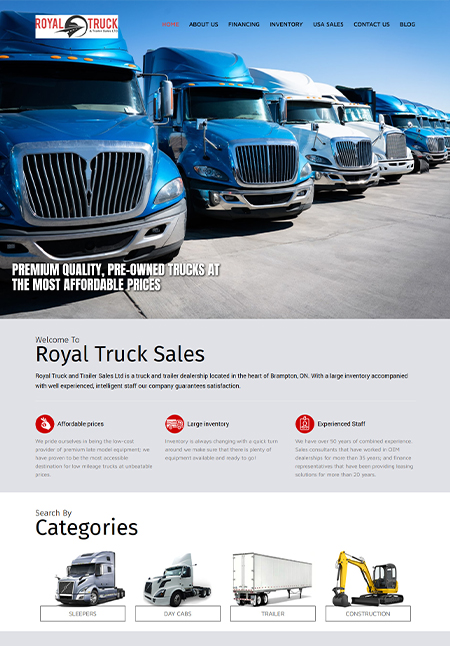The image portrays a website layout that is approximately 50% taller than it is wide. The top half features a prominent banner showcasing a fleet of semi-trucks oriented towards the 4:30 to 5 o'clock position. The trucks are arranged in a descending line from the lower left to the background, totaling around ten vehicles. Most of the trucks are in shades of light to medium blue, with the exception of the third and fourth trucks, which are white.

In the upper left corner of the banner, there is a red "Royal Truck" logo accompanied by a black ship emblem situated between the words. Below this, a tagline reads, "Premium Quality Pre-Owned Trucks at the Most Affordable Prices."

The upper right section displays the main navigation menu, with "Home" highlighted in red and the other options—"About Us," "Financing," "Inventory," "USA Sales," "Contact Us," and "Blog"—in black text.

Beneath the banner, the main content area begins with a welcoming message, "Welcome to Royal Truck Sales," followed by a brief, unreadable blurb. At the bottom of the page, there is a category selection menu for browsing different types of equipment.